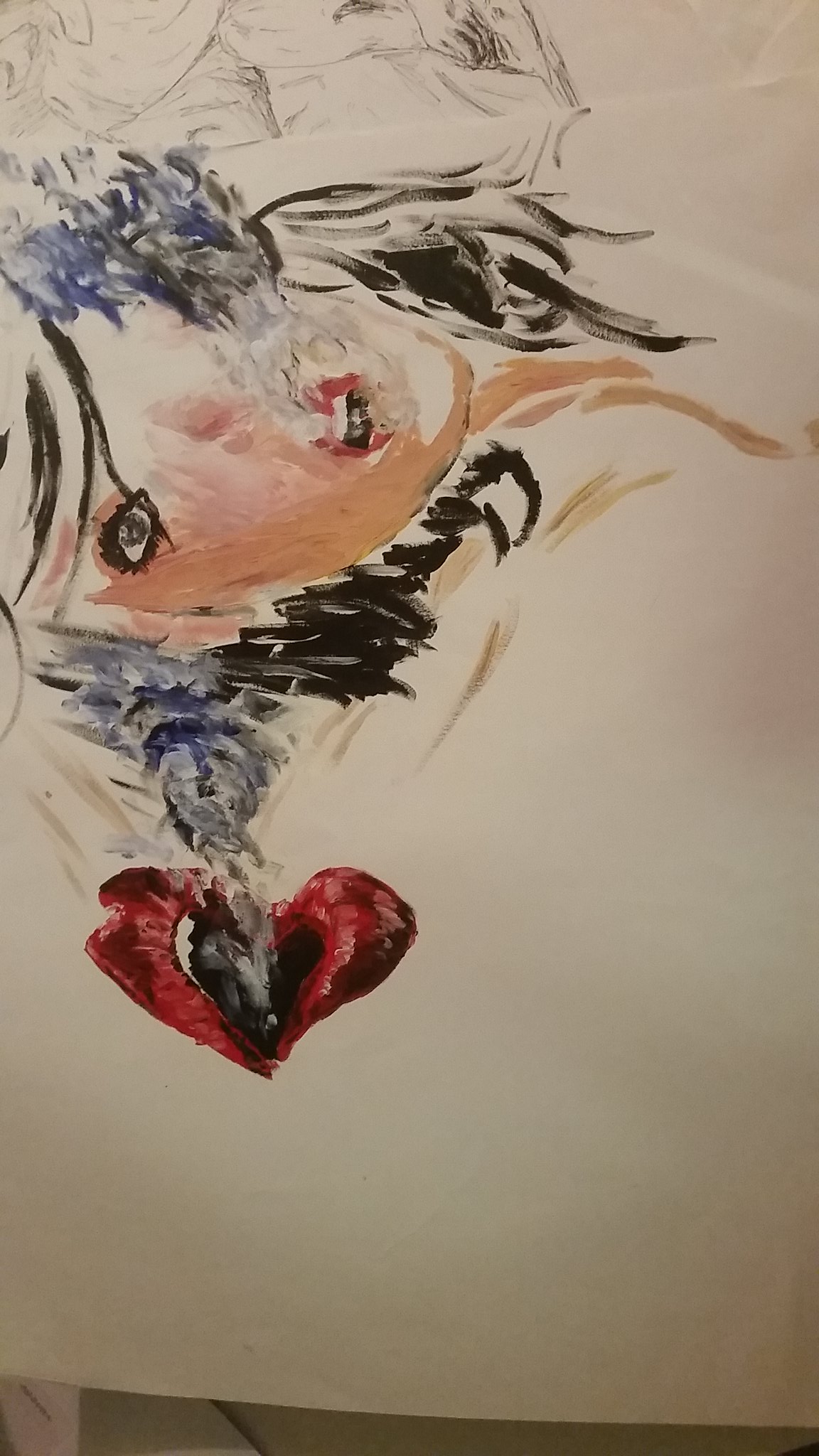This artwork, set on white paper and possibly created with watercolor or a similar medium, features a striking and modern stylistic representation of a woman. The composition is unique as the woman's head is oriented horizontally across the top portion of the image. She dons bold red lips and dark black mascara accentuating her eyes, which starkly contrast her deep black hair. A mysterious blue element is also present behind her, adding a touch of intrigue. Moving towards the middle and bottom sections of the piece, there appears to be a heart shape, further contributing to the abstract and representational nature of the artwork. Rather than aiming for photo-realism, the artist has opted for a contemporary approach to capture the essence and emotional undertones of the female subject.